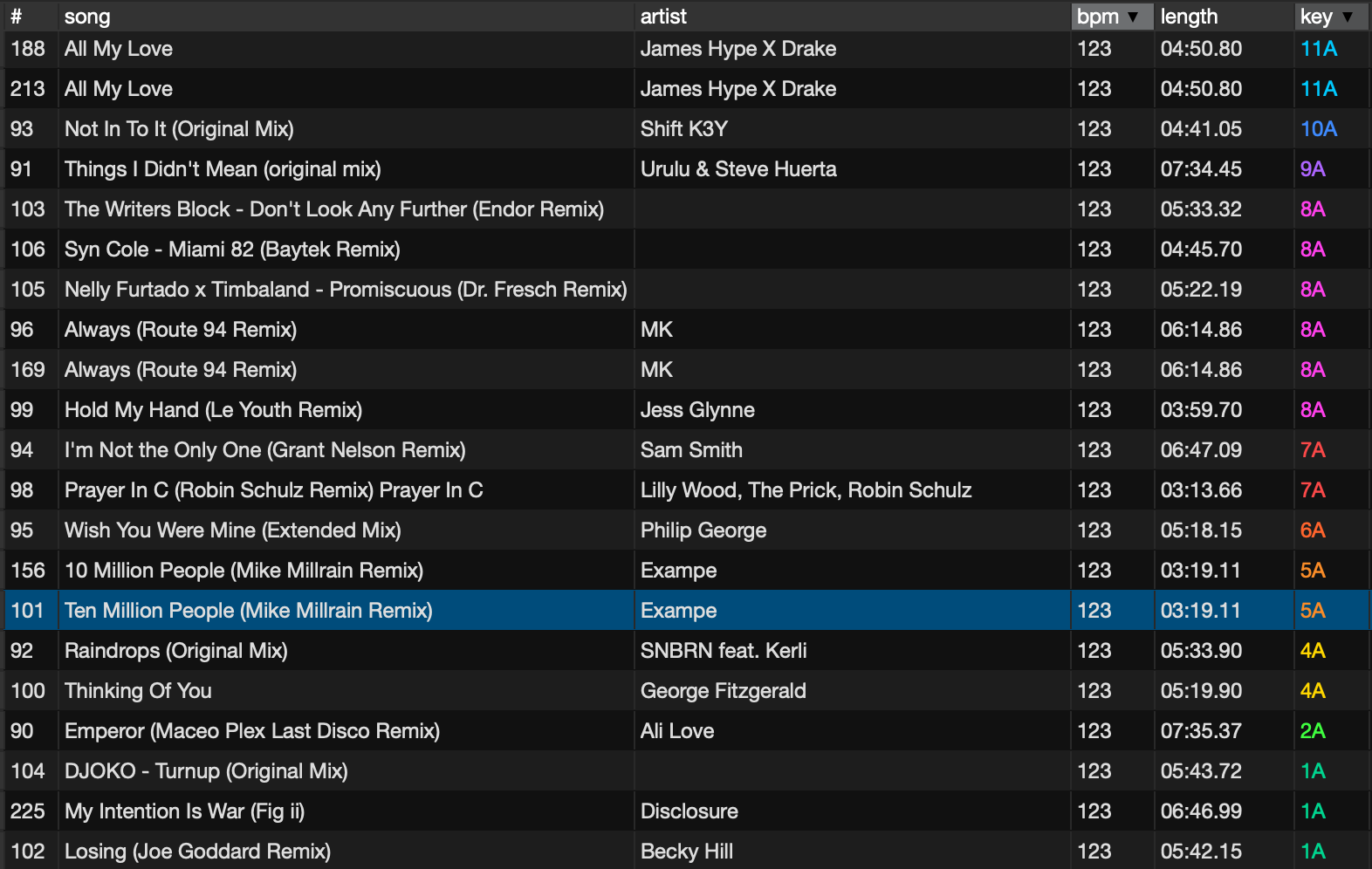This screen capture showcases a music-playing application with a sleek, dark interface, featuring neatly organized information in a grid layout. The background alternates between black and dark gray rows, providing a visual distinction between each entry. The grid consists of six columns, each presenting different attributes of the songs listed.

From left to right, the columns are:
1. **Index**: This column displays numbers that appear in a non-sequential, random order.
2. **Song Title**: Lists the titles of various songs, including multiple occurrences of "All My Love", "Always (Route 94 Remix)", and "10 Million People".
3. **Artist**: Shows the performer of each track, with some entries left blank. Notable artists mentioned are MK, Jess Glynne, and Sam Smith.
4. **BPM (Beats Per Minute)**: Indicates the tempo of the tracks.
5. **Length**: Specifies the duration of each song.
6. **Key**: Features a color-coded system to represent different musical keys, ranging from blue, purple, and pink, to orange, yellow, and green.

All text is displayed in white, except for the Key column, which uses various colors to differentiate between musical keys. This detailed, well-organized layout provides a comprehensive overview of the user's music library, making it easy to navigate and understand.